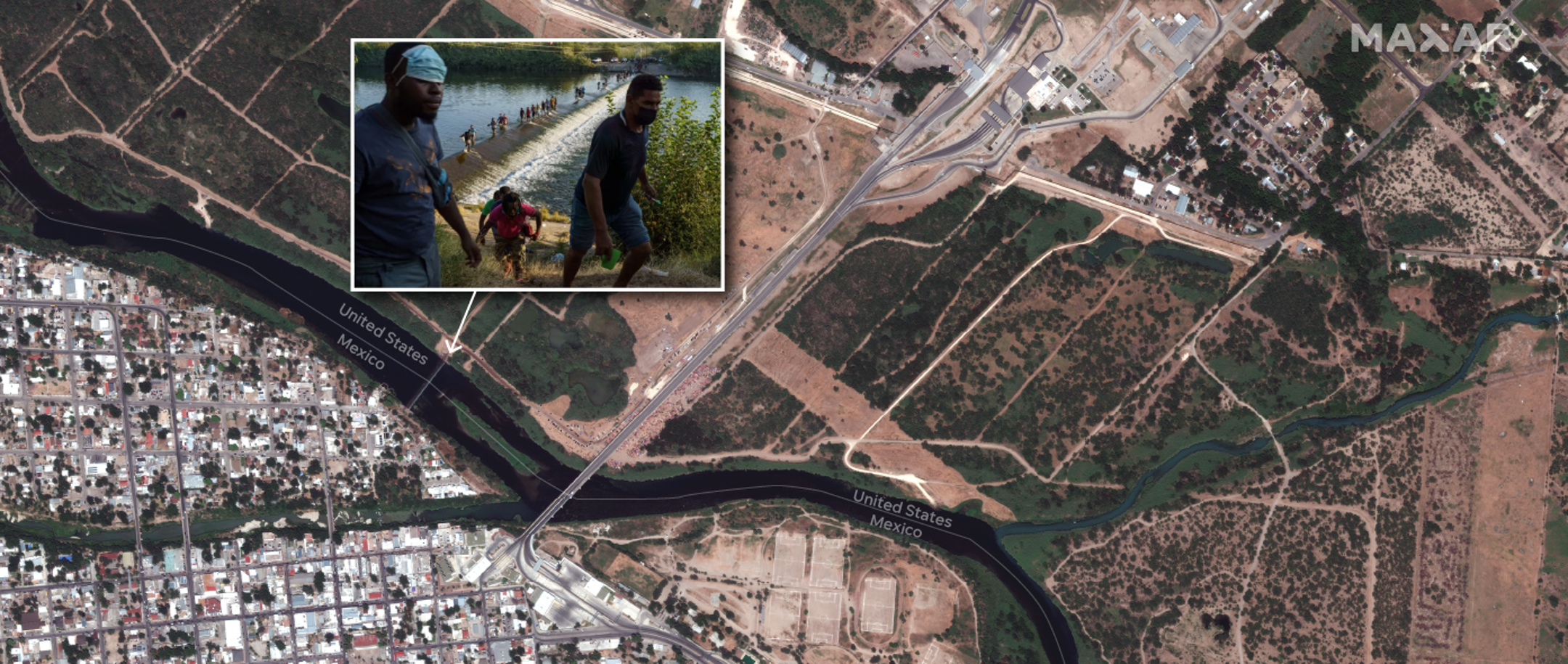The image is an overhead satellite view, possibly from Google Maps, depicting a wide stretch of terrain. The upper part of the image prominently displays the marking "M-A-X-A-R" in a light gray font. In the lower left, there's a residential area characterized by a grid pattern of 90-degree streets and buildings. A black area, likely a river, runs diagonally from the upper left to the middle bottom, delineated by a line that separates the United States and Mexico. 

The terrain varies significantly across the image: the left side shows green patches and rocky brown areas, while more central and right portions reveal alternating regions of greenery, dirt, and roads. One prominent highway traverses diagonally from the bottom left towards the upper middle, intersecting varying landscapes. 

Inset into the larger satellite image, slightly left of center, is a small box bordered in white. Inside this box is a close-up thumbnail of three people walking on the terrain shown in the satellite view. One man wears a blue hat, accompanied by another adult and a child in a red top, against a backdrop of water and greenery. A white arrow beneath the inset image points to their location on the overhead map, linking their position to the expansive landscape.